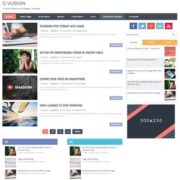The image depicts a highly blurred and miniature screenshot of a webpage with a white main background. At the top of the page, there is a narrow bar containing an indistinct word in the top left corner, followed by some black subtext underneath. Below this, a black navigation bar spans the entire width of the page, featuring eight different tabs. The first tab is highlighted in red, indicating the current section.

Directly under the navigation bar, there are four visible content blocks. Each block contains a rectangular thumbnail on the left, accompanied by a bold heading and some descriptive subtext to its right. At the bottom of these blocks is a pagination section featuring five blocks, one of which is red, signifying the current page out of at least four pages. A "Next" button is also present.

Occupying the right-hand side of the page is a comprehensive navigation menu comprising several small thumbnails with corresponding information and links to various social media pages related to the website. At the bottom of the page, two columns stand out with distinctively colored headings—one purplish blue and one turquoise blue—each displaying three thumbnails beneath them.